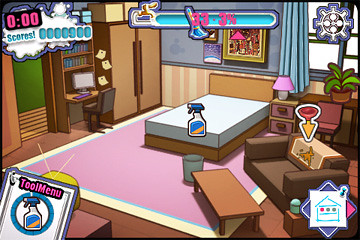This image is a vibrant and detailed screenshot from a computer game set in a colorful, cartoon-style bedroom or studio apartment. The room features a significant baby pink carpet with a white border, which covers almost the entire floor. The main elements include a brown bed with a white mattress, holding a white spray bottle with a blue top. In front of the bed stands a wastebasket, and a nightstand with a pink lamp is positioned to the side. A brown recliner sits next to a coffee table, and behind the recliner is a desk adorned with a chair, a flower pot with a blooming plant, and a computer monitor. 

On the far wall, a cabinet and a bookcase are present, indicating storage. A window with blue curtains provides a backdrop for the desk. A scores display, a health bar, and a tool menu with a cleaning spray bottle are visible on the interface, suggesting that this is a cleaning game. A timer shows zero, and a percentage bar is marked at 33.3%. In the bottom right corner, there's a purple diamond shape with a white square on top, featuring a drawing of a house and a piece of paper, further emphasizing the game's interactive elements. Overall, the room is densely furnished, resembling a cozy dorm room or a bachelor’s studio, designed with a lively, animated aesthetic.